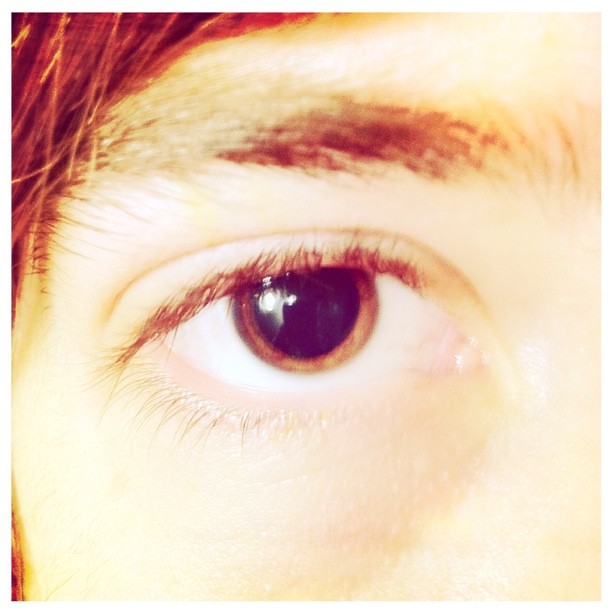This image depicts an extreme close-up of a person's right eye. The individual appears to be Caucasian with brown hair, making them likely a brunette. Their eye is a striking brownish amber, with a large, dilated pupil. The surrounding sclera is white, and the reflection in the pupil reveals a person holding up a camera phone, suggesting that this image was taken in an indoor setting with controlled lighting. The person has double eyelids, which seem a bit droopy, possibly indicating hooded eyelids. Their eyebrow is brown and somewhat sparse in the beginning half but becomes denser towards the end. The presence of slight bags under the eye hints at a young age. Additionally, the image features a noticeable orange filter that enhances the warm hues of the photograph. You can also see a portion of the person's head and the edge of their nose in the frame.